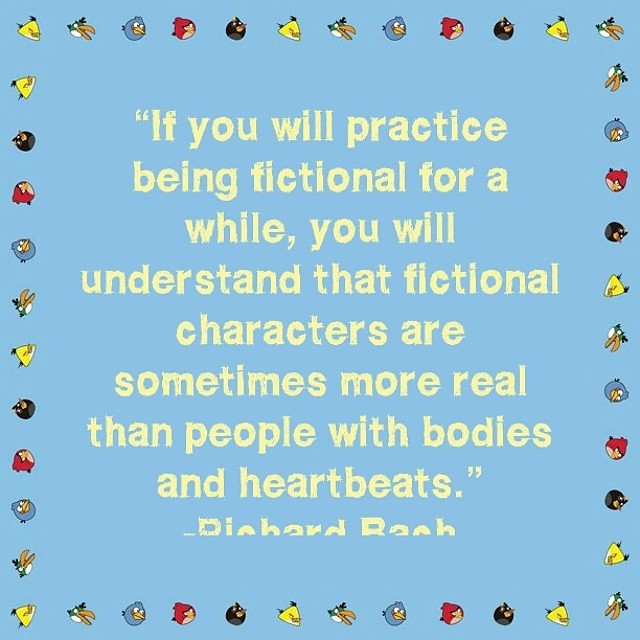The image features a square layout with a light sky blue background. In the center, a quotation in pale yellow lettering reads, "If you will practice being fictional for a while, you will understand that fictional characters are sometimes more real than people with bodies and heartbeats." The author of the quote, Richard Bach, is partially visible, with half of his name obscured. Surrounding the quote, the border is adorned with a variety of colorful little heads from the Angry Birds game, approximately 12 per side, adding vibrant reds, blacks, yellows, blues, and other hues that contrast nicely with the dull blue background.